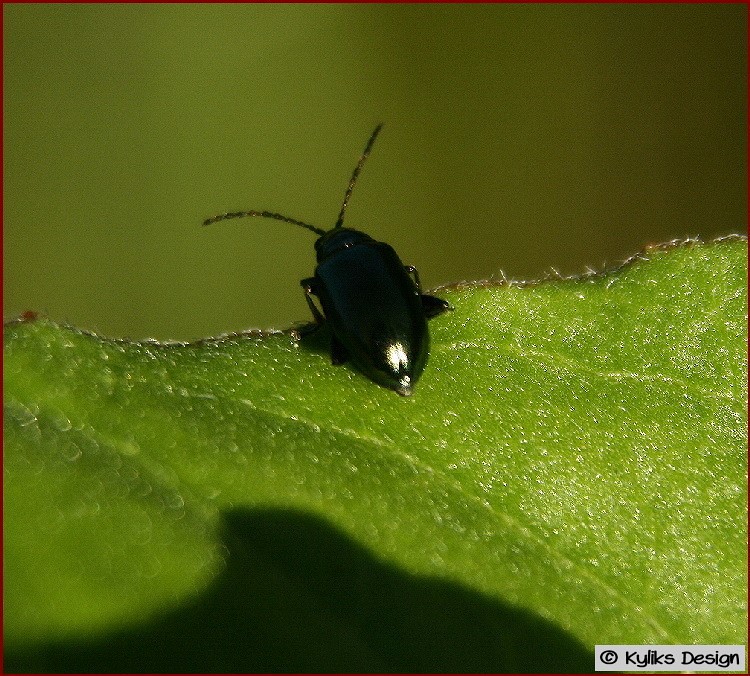The photograph captures a close-up of a small, black, shiny beetle perched on the serrated edge of a green leaf. The leaf forms the entire bottom half of the image and is brightly illuminated, suggesting an outdoor, daytime setting. The beetle, approximately half an inch or smaller in size, faces away from the camera, showcasing its smooth, shell-like back and long, curved antennae with black and tannish-gray hues. The background of the upper half of the image is a blurred, dark green, enhancing the focus on the insect and leaf. The photograph bears a copyright mark that reads "Kylix Design" in the bottom right corner, indicating the photographer. The image exemplifies detailed wildlife photography.